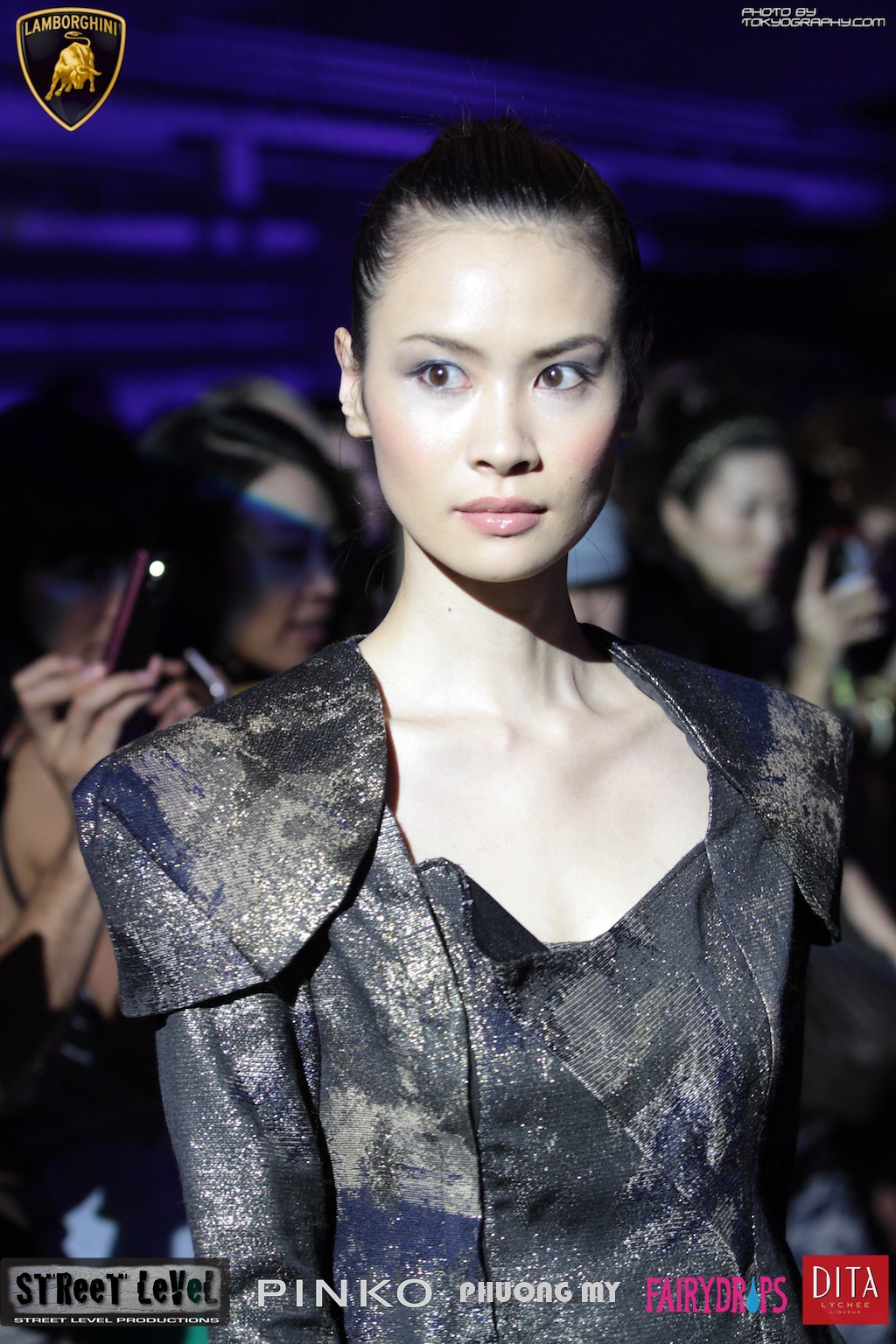In this captivating photograph, an elegant model with tightly pulled back dark hair and a serene, almost serious expression, gazes off into the distance. She is wearing a glittery, dark charcoal dress with splotchy, paint-like patterns that shimmer, creating a striking visual contrast. The model exudes an air of effortless grace and beauty, enhanced by her mild makeup that highlights her delicate features, suggesting she may be of Asian descent.

The background is filled with out-of-focus spectators, all holding up their cell phones to capture the moment, adding to the atmosphere of an exclusive event. The bottom of the image is adorned with sponsor logos including Street Level, Pinko, Fairy Drops, and Dita. Additionally, a Lamborghini logo appears at the top left, and a watermark on the right side reads "photo by TOKYOGRAPHY.COM", suggesting a high-quality, professional composition. This powerful image encapsulates the glamour and allure of a high-profile fashion event.